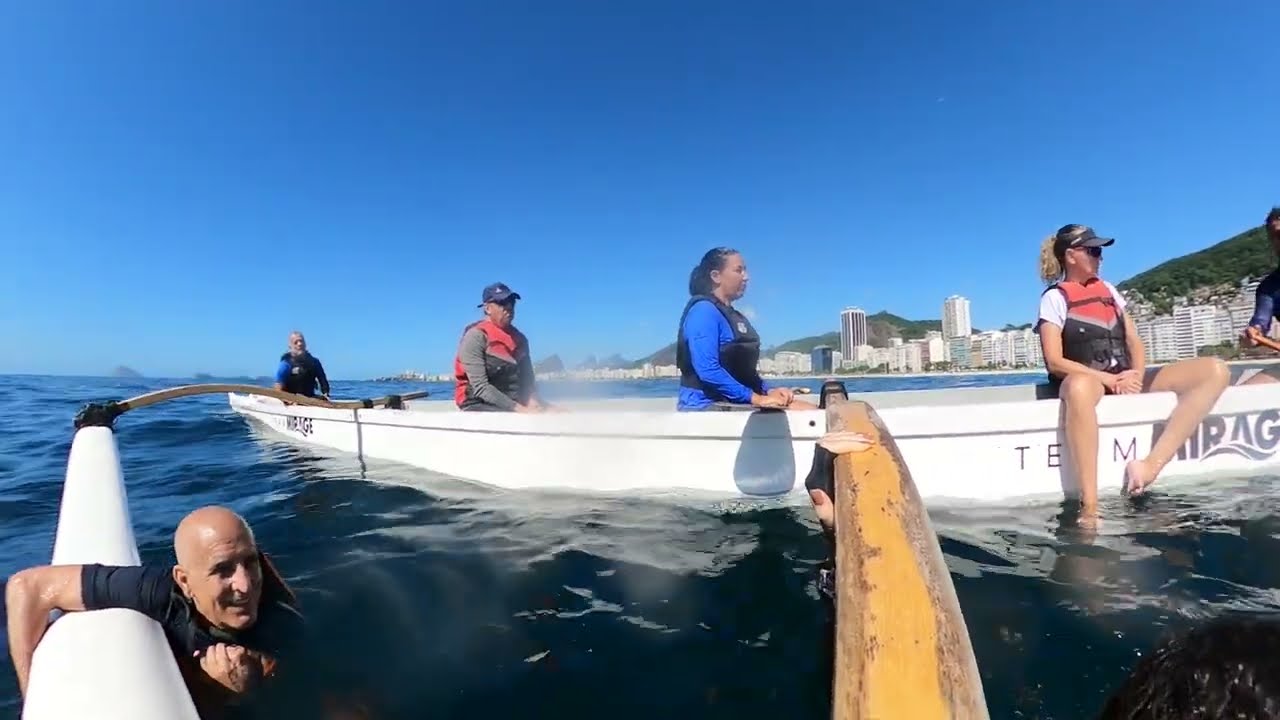In this vibrant outdoor image taken from within a body of water, a large, white boat reminiscent of a pontoon or a kayak is prominently featured. The boat, which has sleek, long extensions resembling pontoons or wooden platforms, accommodates around five seated passengers, both men and women, all wearing safety jackets. The boat’s letters “T-E-M-M-I-R-A-G” are clearly visible in black paint along its side. Additionally, there are two people in the deep blue water holding onto the boat's strings or extensions, one of whom is a bald man smiling. The scene is bathed in daylight under a cloudless, light blue sky. In the distance, the coastline is dotted with numerous hotels and buildings, adding an urban backdrop to this serene aquatic adventure.